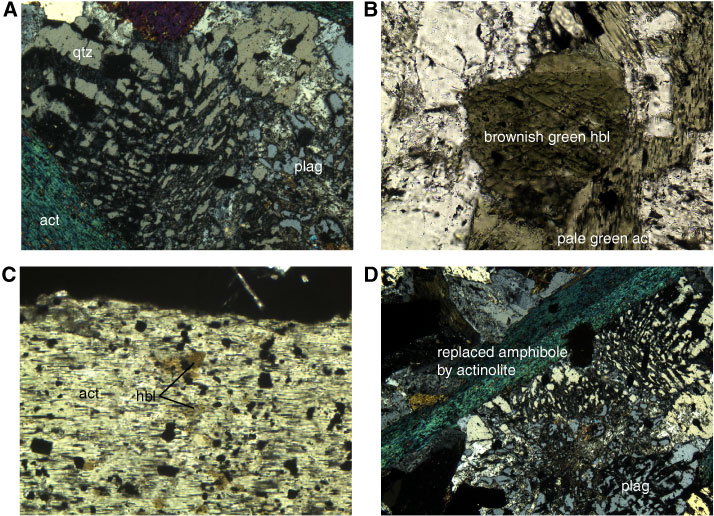The image comprises a grid of four smaller images labeled A, B, C, and D, each depicting different types of rocks with distinct colorations and labeled details. Image A features a predominantly grayish rock with a sponge-like texture, labeled "QTZ," "ACT," and "PLAG," with a brownish-green corner section. A text label on this image reads "Plagg." Image B shows a rock in various shades of green, labeled "brownish green HBL" and "pale green ACT," with dark black markings throughout. Image C presents a yellowish rock marbled with black spots, labeled "ACT HBL." Finally, Image D displays a rock similar in color to Image A, marked with the text "replaced amphibole by actinolite." All text appears in a sans-serif font, enhancing readability.